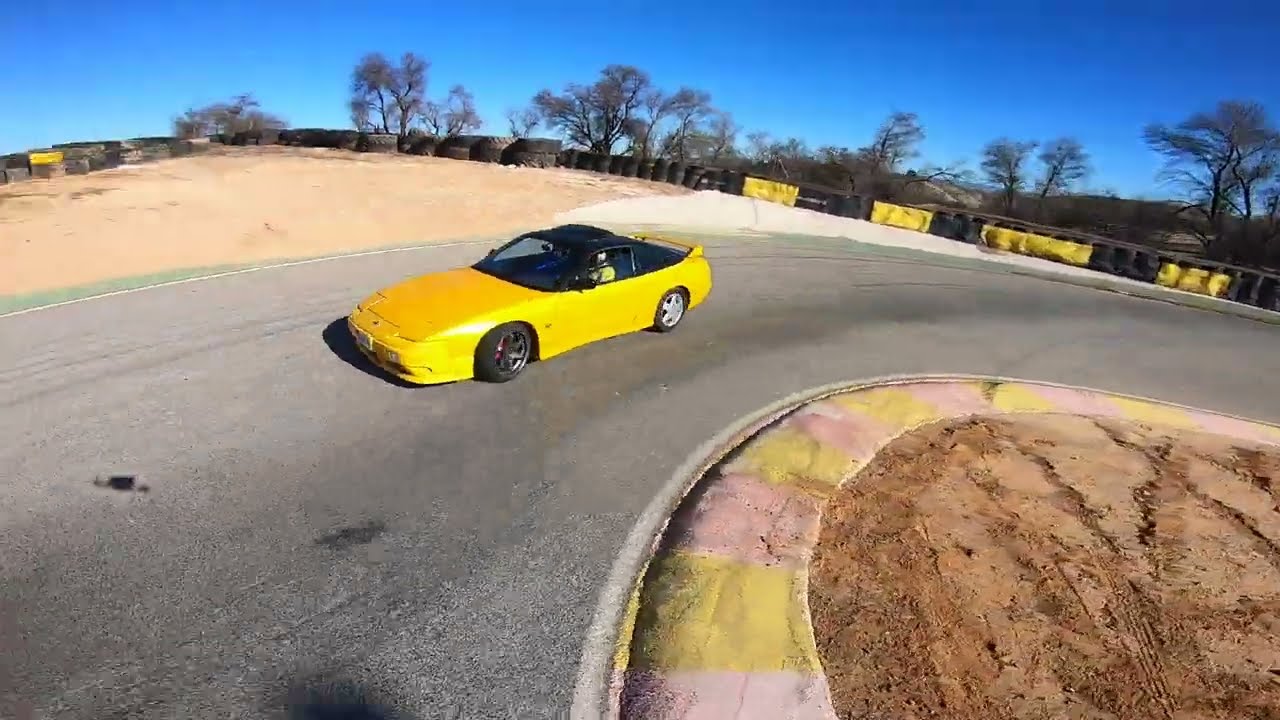The image showcases a yellow sports car with a black top, navigating a curved car racing track that extends from the right side of the image, curves in the center, and continues to the bottom left. The car, driven by a visible person and equipped with red brake calipers, a sunroof, and a spoiler, is captured mid-turn to the left. The racetrack features distinctive pink and yellow-striped concrete borders, with red clay dirt in the middle section and additional yellow banners decorating a wooden fence on the left side of the path. Behind the fence, trees with sparse foliage stretch diagonally along the horizon. The bright blue sky and shining sun suggest that the scene is set during the daytime, possibly in the afternoon, away from urban areas, potentially in a desert or sand dune region.